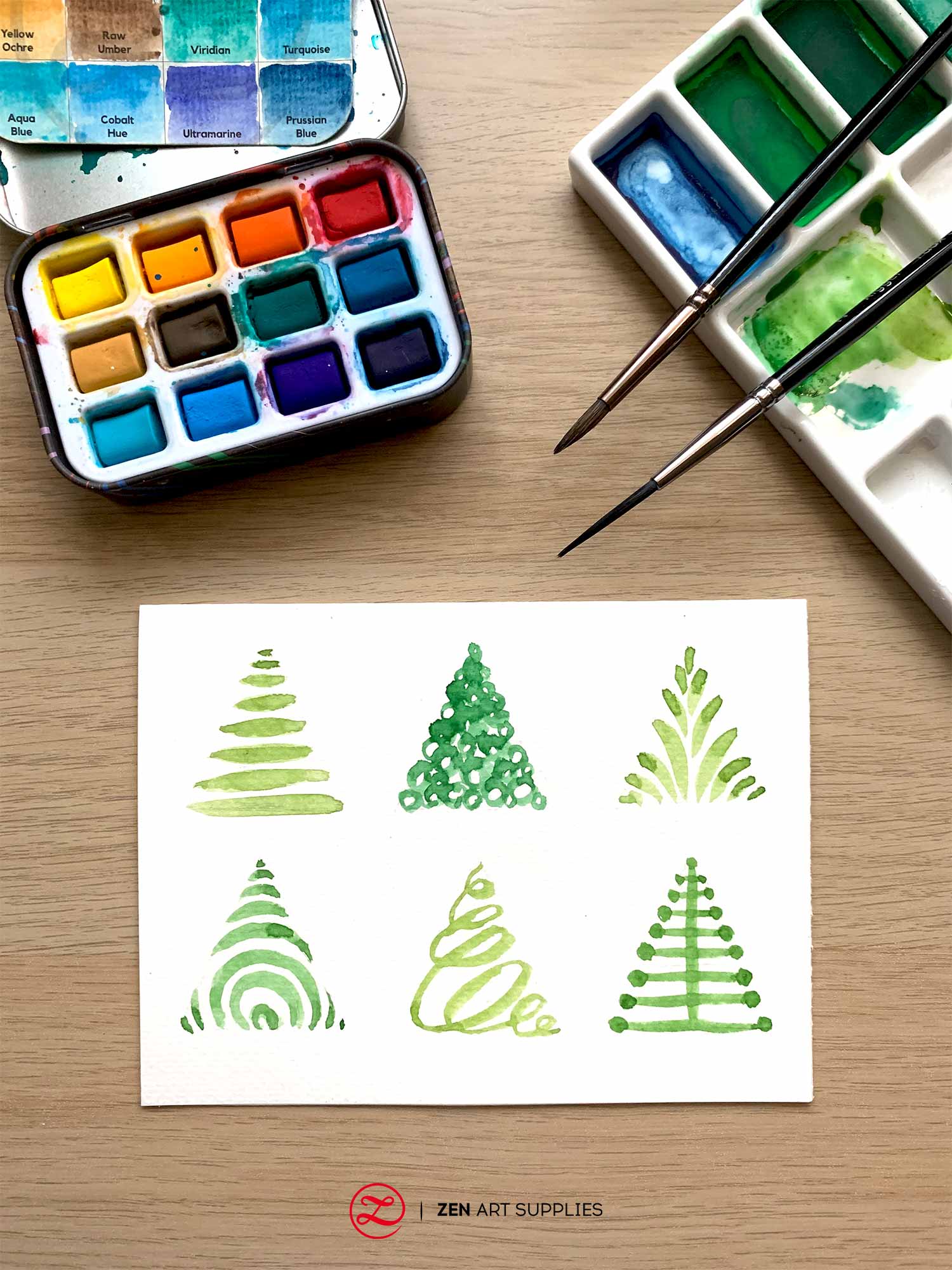This image captures a vertically aligned rectangular photograph that looks down on a medium brown, finely grained desk or table surface. Centrally towards the bottom lies a horizontally placed piece of white drawing paper or cardstock, adorned with various painted images of green trees, resembling Christmas trees in different forms such as layered, clustered, and featuring long sprouting leaves and curly branches. In the upper right corner, there is a large tray containing various paints and two slim paintbrushes hanging off it, with a noticeable amount of green paint. In the upper left corner, another tray contains twelve messy-looking watercolors in the shades of red, orange, gold, yellow, light brown, black, forest green, blue, teal, bright blue, indigo, and navy blue, possibly finger paints. At the bottom center, the words "Zen Art Supplies" are inscribed, completing the artistic setup.